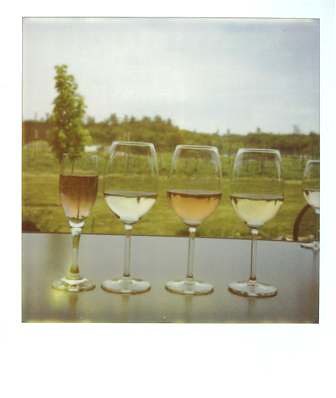The image appears to be an old, faded photograph, offering a nostalgic glimpse into a tranquil outdoor setting. The background showcases a serene countryside under a sky painted with a grayish-blue hue, dotted with wispy white clouds. Below the sky, a diverse treeline of varying heights and shades of green frames the scene, leading down to a well-manicured lawn with short grass. A slight hill with a tall, leafy, yet slender tree is visible on the left side.

In the foreground, a long black or brown table is adorned with five distinct glasses. Four of these glasses are neatly aligned in a row, while the fifth glass is positioned diagonally up and to the right. Among the glasses, three are wide-bodied wine glasses, and one is a slender champagne flute. The champagne flute contains a darker liquid, nearly filling three-quarters of the glass, while the others each hold beverages of various hues—light almost clear, tan, and white—each with a small layer of a solid black substance floating atop the liquid. This vivid yet intimate scene evokes a sense of leisurely elegance amid a picturesque rural backdrop.